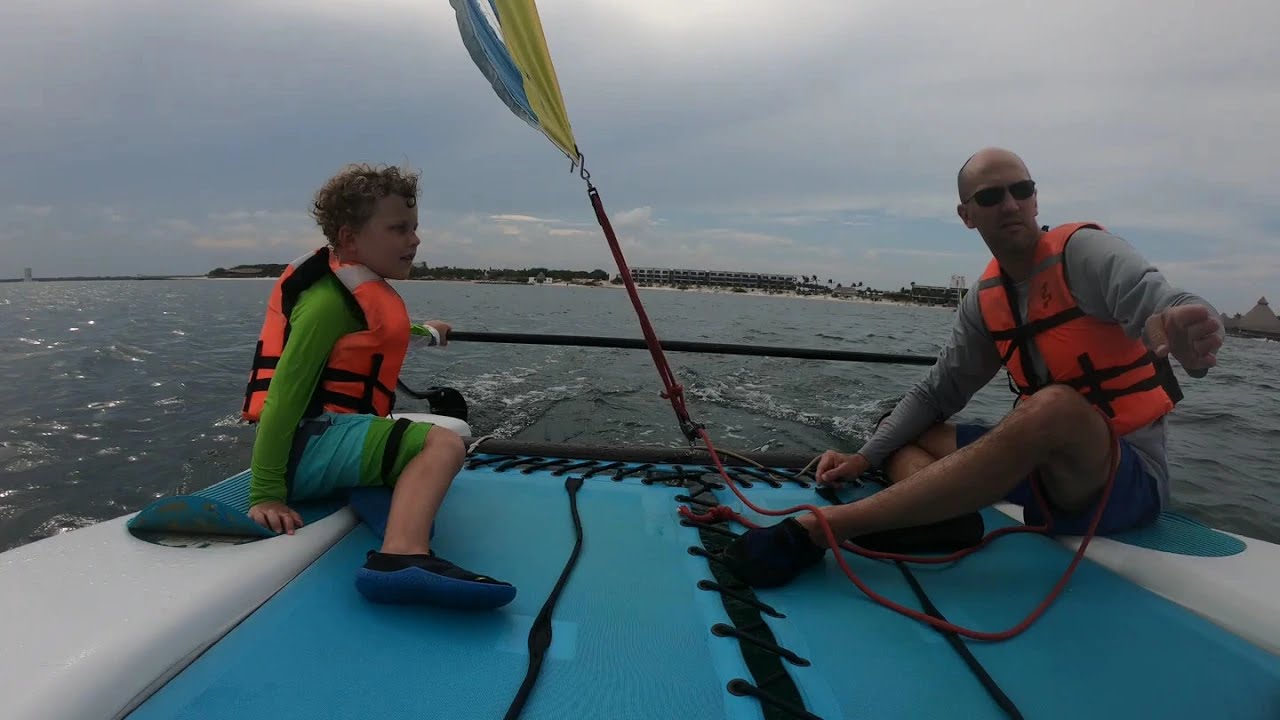In this image, a boy and an adult male, possibly his father, are positioned on the edge of a moving boat, likely a sailboat or catamaran. The boy, seated on the left, appears to be around 8 or 9 years old and is dressed in an orange life jacket, a green and blue swimsuit, and blue shoes. The adult male, on the right, is wearing sunglasses, an orange life jacket, a gray long-sleeve shirt, blue shorts, and black shoes. Both are sitting on a blue canvas-like material that partially covers a harder white section of the boat. The boat is in motion, indicated by the wake pattern in the water behind them. A rope with cloth material, part of the boat's sail setup, runs between the two. In the far background, there's a flat landmass with some vegetation, and possibly a glimpse of a resort or hotel. The sky is fairly cloudy, suggesting either an overcast day or a time shortly before evening.